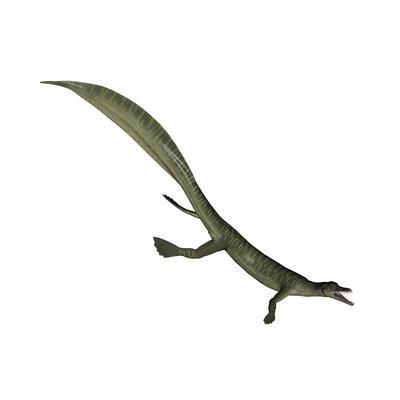The image showcases a digital rendering of a juvenile alligator against a plain white background. The young reptile features a blend of green and tan hues, with its body displaying characteristics that set it apart from a fully-grown alligator. The most notable difference is the tail, which is exceptionally long and wide, resembling that of a manatee. Additionally, the back legs are broad and webbed like paddles, while the front right leg is less webbed and more typical of a lizard's limb. The alligator appears to be in a swimming motion, moving downwards to the right. The photograph emphasizes the developing nature of this prehistoric-looking creature, with its tiny head, limited visibility of teeth, and a body proportionally smaller than its prominent tail.